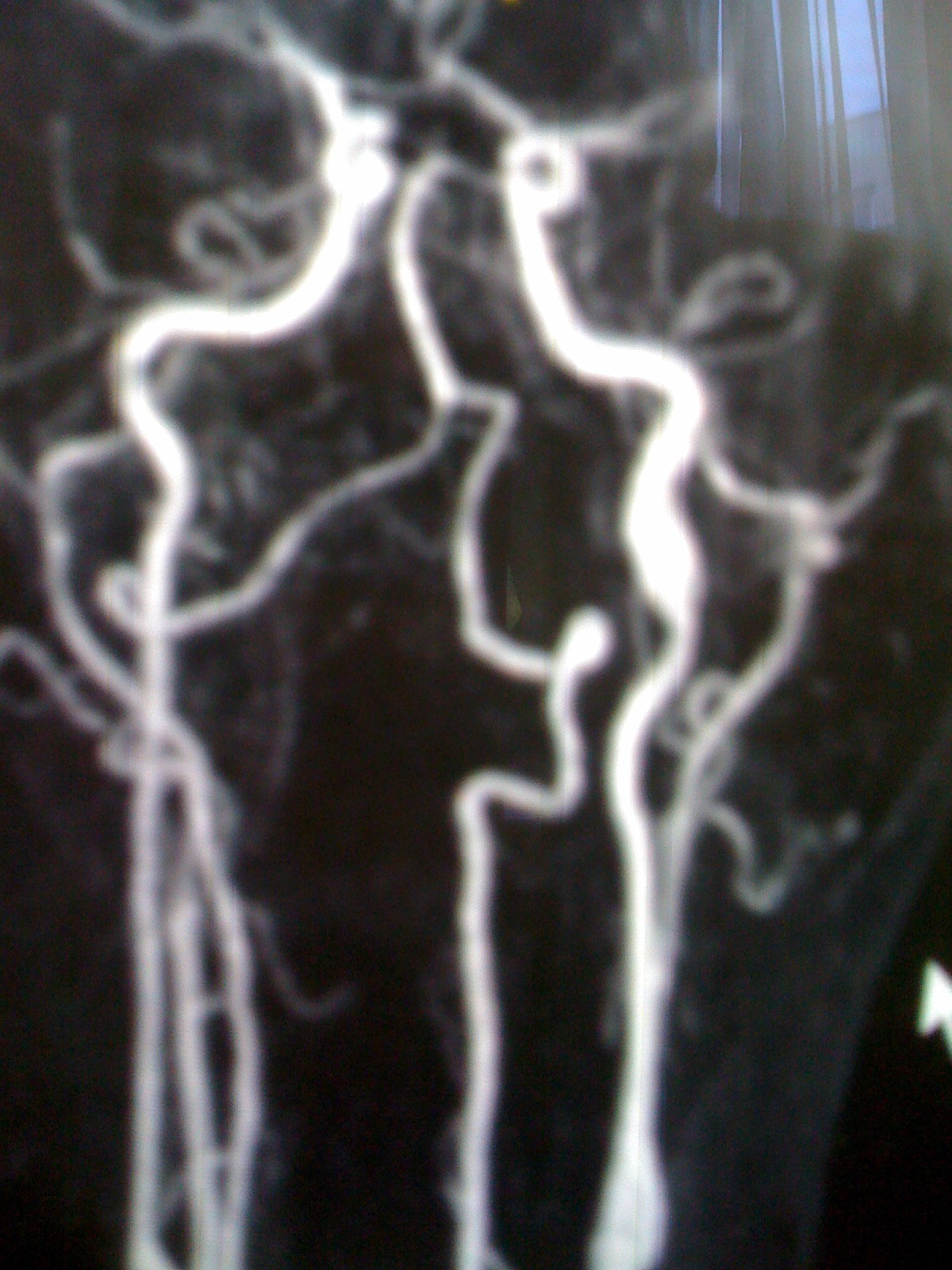This image is out of focus and somewhat abstract, giving the appearance of illuminated, tangled strands resembling a cluster of noodles. The light is intensely bright and seems to function as a light source, casting a stark contrast against the darker areas. These "noodles" vary in thickness and length, creating a dynamic, almost chaotic pattern reminiscent of wriggling worms. In the top right corner of the image, a gauzy curtain partially covers a window, adding a subtle texture and a sense of depth to the composition. The interplay between the bright, noodle-like elements and the surrounding shadows creates an intriguing, mysterious ambiance.